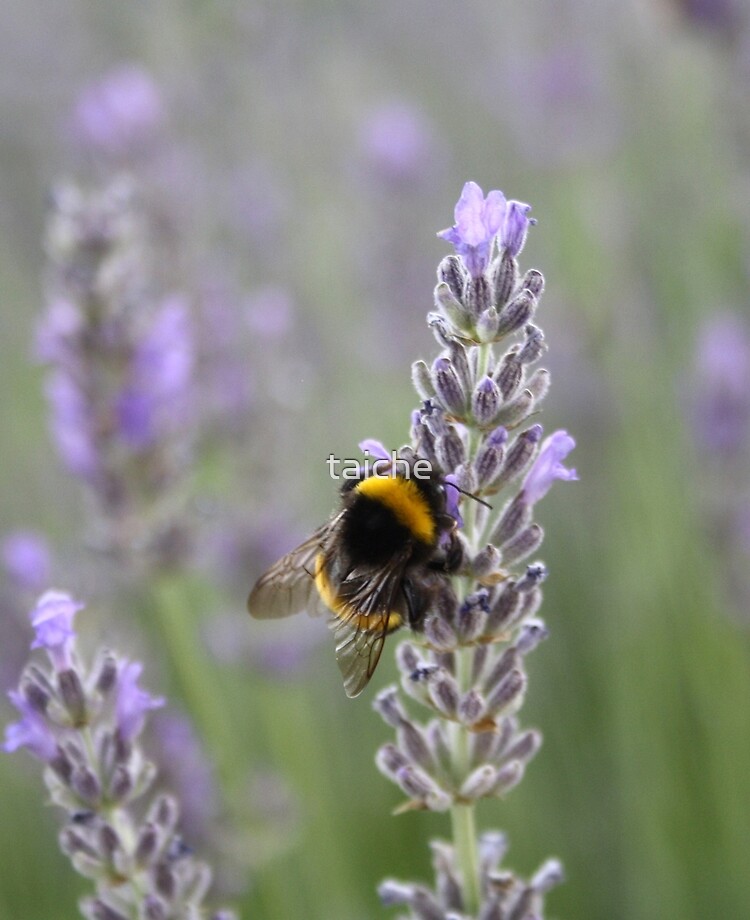This is a detailed close-up nature photograph taken in a field featuring tall lavender plants with partially opened light purple buds. The primary focus of the image is a large, vividly colored bumblebee with brilliant yellow and black stripes, and detailed, translucent wings. It is at the foreground, resting on the flower facing the viewer, where it appears to be extracting nectar or pollen. The background includes more lavender flowers, gradually becoming more blurred, creating a depth-of-field effect. The photograph also includes a watermark in the center, displaying the text "TAICHE" in white, transparent letters, possibly indicating the name of the flower or serving as a signature. The primary colors in the image are shades of lilac and green, with the vibrant yellows and blacks of the bee adding contrast.